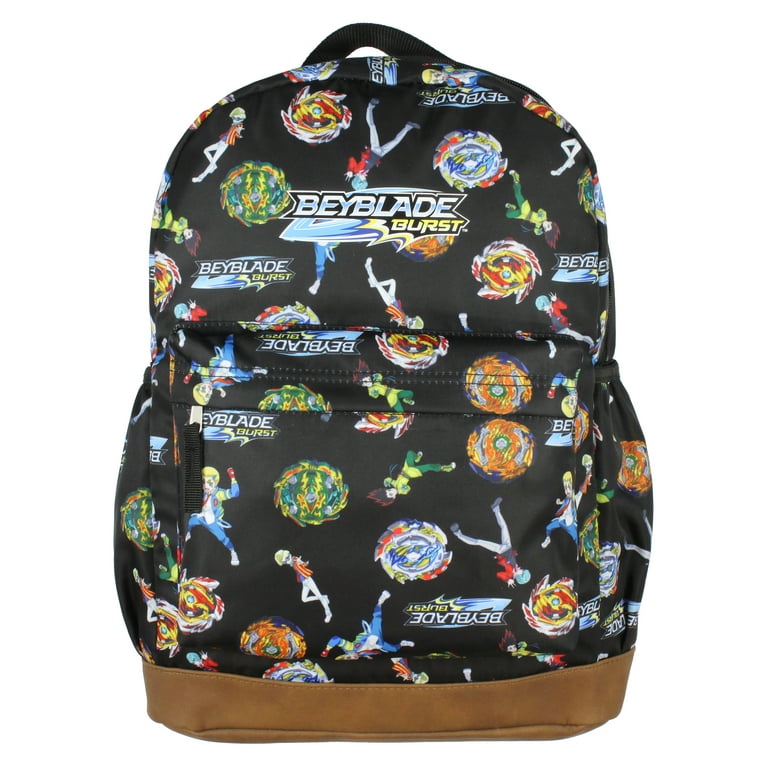The image shows a children's backpack set against a clean, white background. The backpack itself is predominantly black with a gray suede bottom, but it has a broad array of vibrant designs. It features various dynamic figures and symbols related to the Beyblade Burst series. Prominently displayed at the center is the text "Beyblade" in silver and "Burst" in yellow. The backpack's design includes multiple circular motifs resembling Beyblades, each colored distinctively—green, blue, red, orange with blue and white swirling flames, and more mixtures of blue and yellow. Among the dynamic figures, one character with blonde hair, a blue outfit, a white shirt, and a red glove appears to be cheering, while another is lying on their back, wearing white pants and a yellow and red shirt. There's a top handle, albeit black, for carrying or hanging. The backpack's front zipper is visible, though partially obscured by the intricate, scattered designs that cover the entirety of the backpack, making it a lively, eye-catching accessory appropriate for a child.